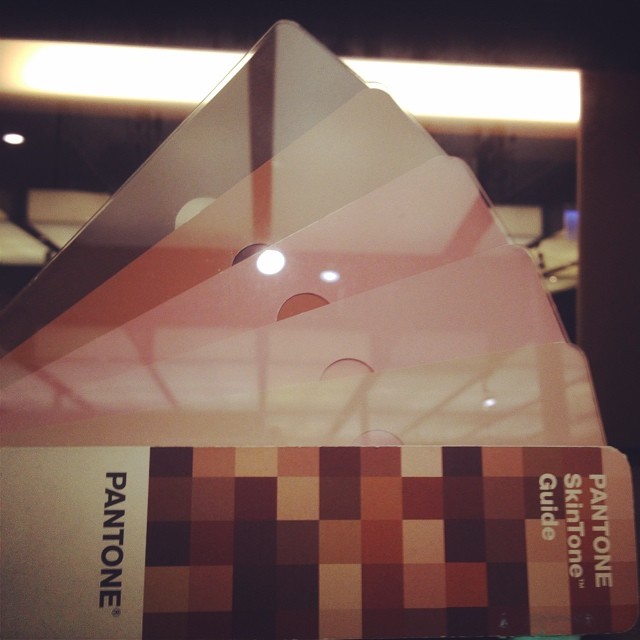This square-format photograph presents a detailed and clearly composed Pantone Skin Tone Guide. Central to the image is a horizontally situated cover that reads "Pantone Skin Tone Guide" in white letters on a checkerboard pattern of browns, grays, and whites, with the word "Pantone" boldly set in black to the left. The cover is partially overlaying a neatly fanned-out array of five color swatch sheets, ranging from beige to light pink, darker pink, reddish-brown, and finally a darker brown. Each sheet features a distinct central cut-out hole. The setting appears to be indoors, with reflections hinting at glass protection over the guide. The background reveals a softly lit room, evident by a white or yellow overhead light and architectural elements like a door frame, providing a context that enhances the primary focus on the color guide itself.